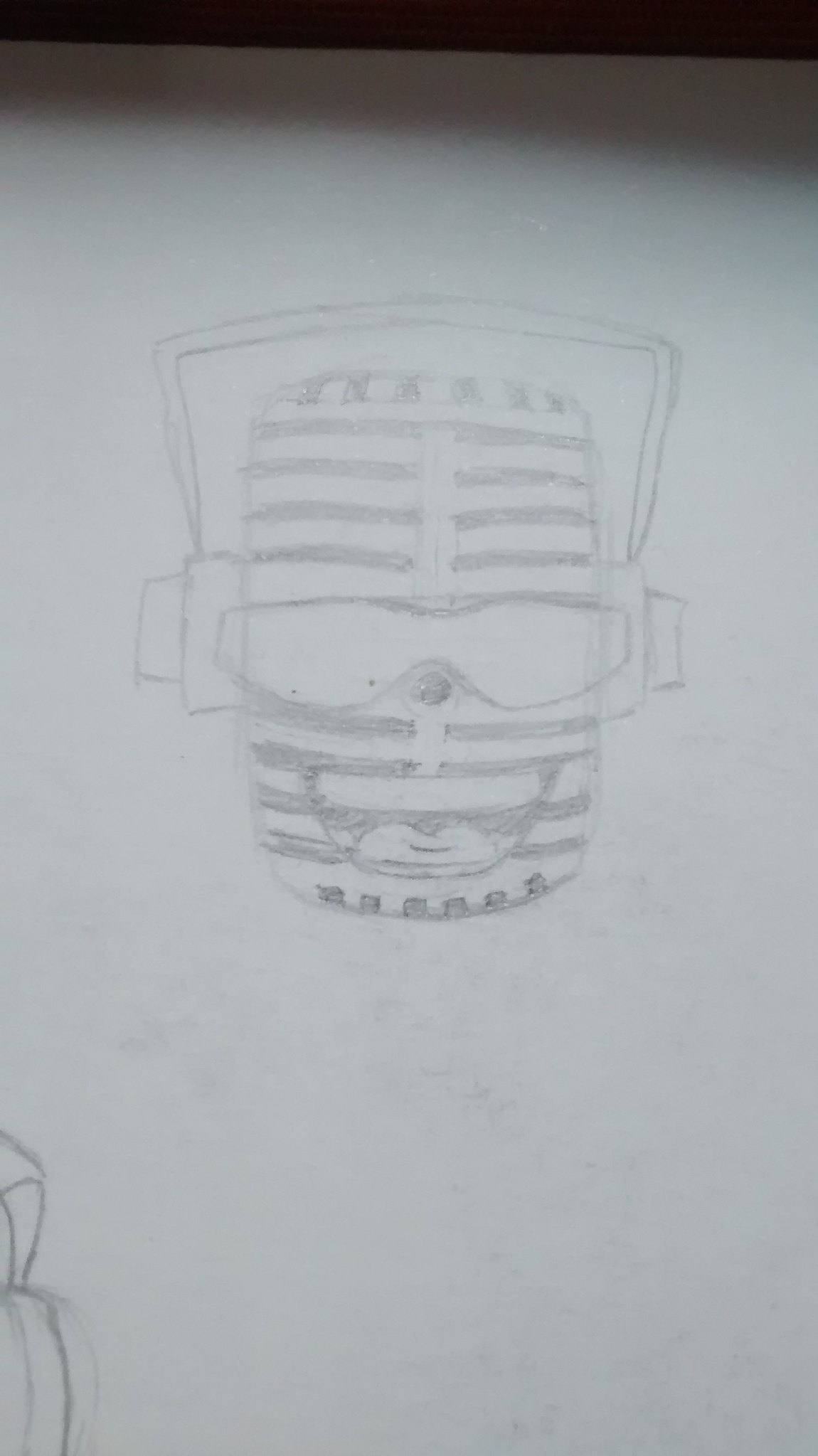This detailed pencil sketch depicts the face of a humanoid character. The artwork focuses solely on the face, with the exception of a few sketch lines in the lower left-hand corner. The head is adorned with a distinctive pair of headphones, which are square-shaped and extend upwards before ending in double circular pads that presumably cover where the ears would be. The figure also sports glasses, a rounded nose, and a mouth with a visible tongue. The entire sketch is rendered in shades of grey on a white background, typical of pencil artistry. Intriguingly, the face is horizontally striped from the forehead down to the chin, while the chin and the very top of the head are marked with vertical stripes, adding unique dimensionality to the character's design.